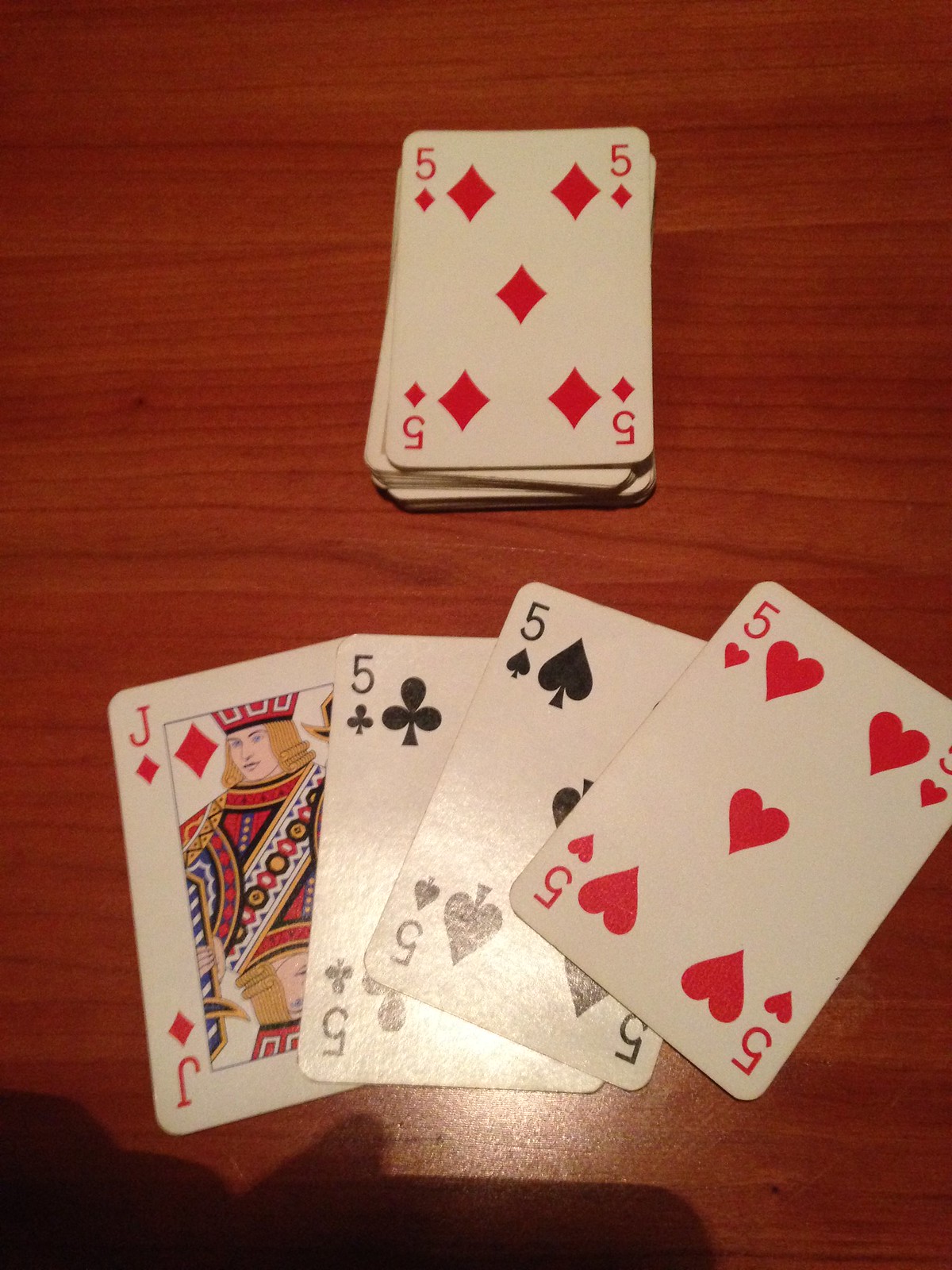This photograph features an arrangement of poker playing cards spread out on a wooden table with distinct black and cream streaks, enhancing the authentic wood texture. At the top of the image, a small deck of cards is partially visible, with the five of diamonds prominently displayed as the top card, showcasing its trademark red diamonds and '5' numerals in all four corners.

Positioned horizontally beneath this deck, four individual cards are laid out side by side. They are, from left to right: a red joker card, a black five of clubs, a black five of spades, and a red five of hearts. The red joker card, with its characteristic vibrant design, stands out against the more conventional playing cards. Subtly, the bottom left corner of the image reveals the soft silhouette of the photographer's shadow, adding a candid element to the scene.

The composition of the cards, coupled with the rich texture of the wooden table, creates an intriguing visual narrative of a paused moment amidst a game of poker.